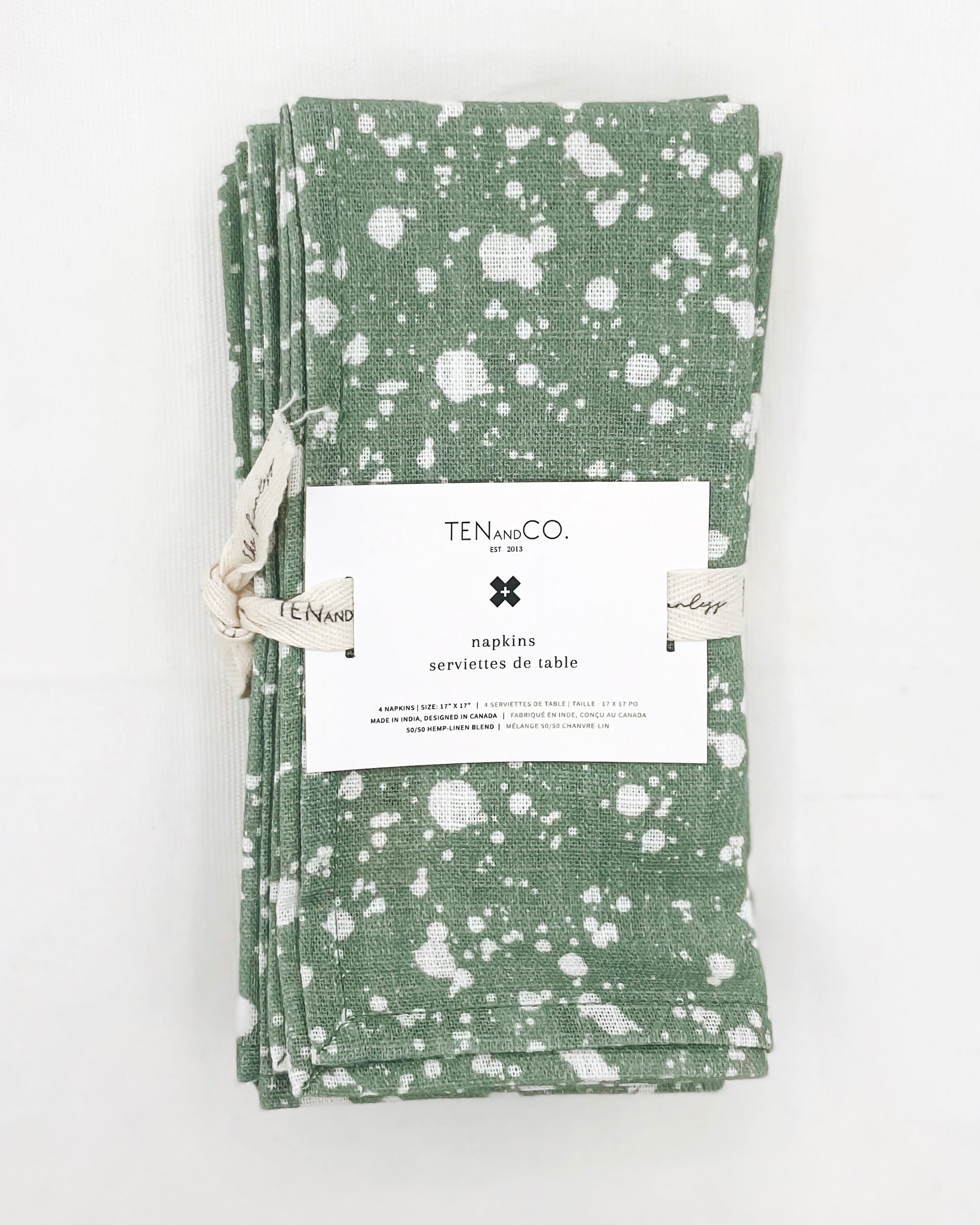This photograph features a neatly wrapped bundle of green cloth napkins adorned with white specks. The napkins are tied together with a white ribbon, adding to their presentable appeal. The packaging includes a label from "Ten & Co.," marked by a distinctive black logo featuring four small diamonds and a central white cross, likely forming an X shape. The label is prominently placed and contains smaller, harder-to-read text likely detailing the product description. The napkins are meticulously folded lengthwise and stacked atop each other, showcasing their uniform design. This detailed image highlights the arranged napkins against what appears to be a white background, making the product's features stand out.